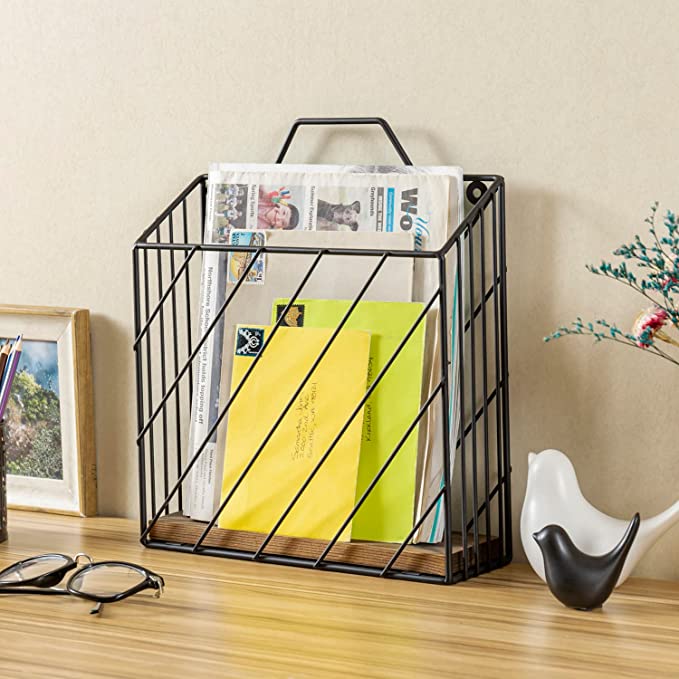This indoor photograph captures a neatly organized desk scene with several distinct objects. At the bottom, the desk features a striped beige wooden surface with a glossy finish. Behind the desk is a slightly mottled beige wall, creating a neutral background. On the far left, leaning against the wall, is a wooden-framed painting in an impressionistic watercolor style, depicting green leaves against a blue sky. In the bottom left corner of the desk, there is a pair of black horn-rimmed glasses folded neatly.

The primary focus of the image is a vertical wire basket made of black metal rods set at 45-degree angles, situated centrally on the desk. This basket serves as a letter organizer and contains a worn newspaper along with three envelopes of varying sizes. The envelopes feature handwritten addresses and black stamps; one contains a white sign, while another has a gold design. Adjacent to the basket, on the right side, are two simplistic bird statues: a larger white bird looking upwards and a smaller black bird in front, looking to the left.

Additionally, a purple pencil can be seen protruding from the left side of the frame, adding a subtle pop of color to the composition. The scene is well-arranged and has a serene, organized aesthetic, capturing everyday items in a thoughtfully curated way.